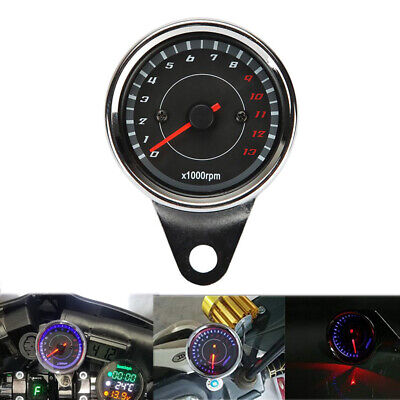The image showcases a central gauge, resembling a speedometer or tachometer, which reads from 0 to 13 with markings indicating 1000 RPM intervals. The numerals from 0 to 8 are displayed in white, and 9 to 13 are in red. A bright red needle points precisely at the zero mark. This central gauge is designed with a stainless steel finish, and at the very bottom, the notation "x1000 RPM" is visible, confirming that each number represents 1000 RPMs. Below the main gauge, there are three smaller images showing the same type of gauge in various applications. The leftmost image appears to show the gauge within a non-automotive vehicle, possibly a plane due to surrounding instrumentation. The middle image depicts another type of vehicle, whereas the rightmost image presents the gauge in a dark setting with the red indicator glowing. The numerals on these smaller gauges are difficult to discern. Additional numbered labels such as 412, 0, 24, and 39 can also be seen on the leftmost image, providing more context or settings related to the gauge's operation.